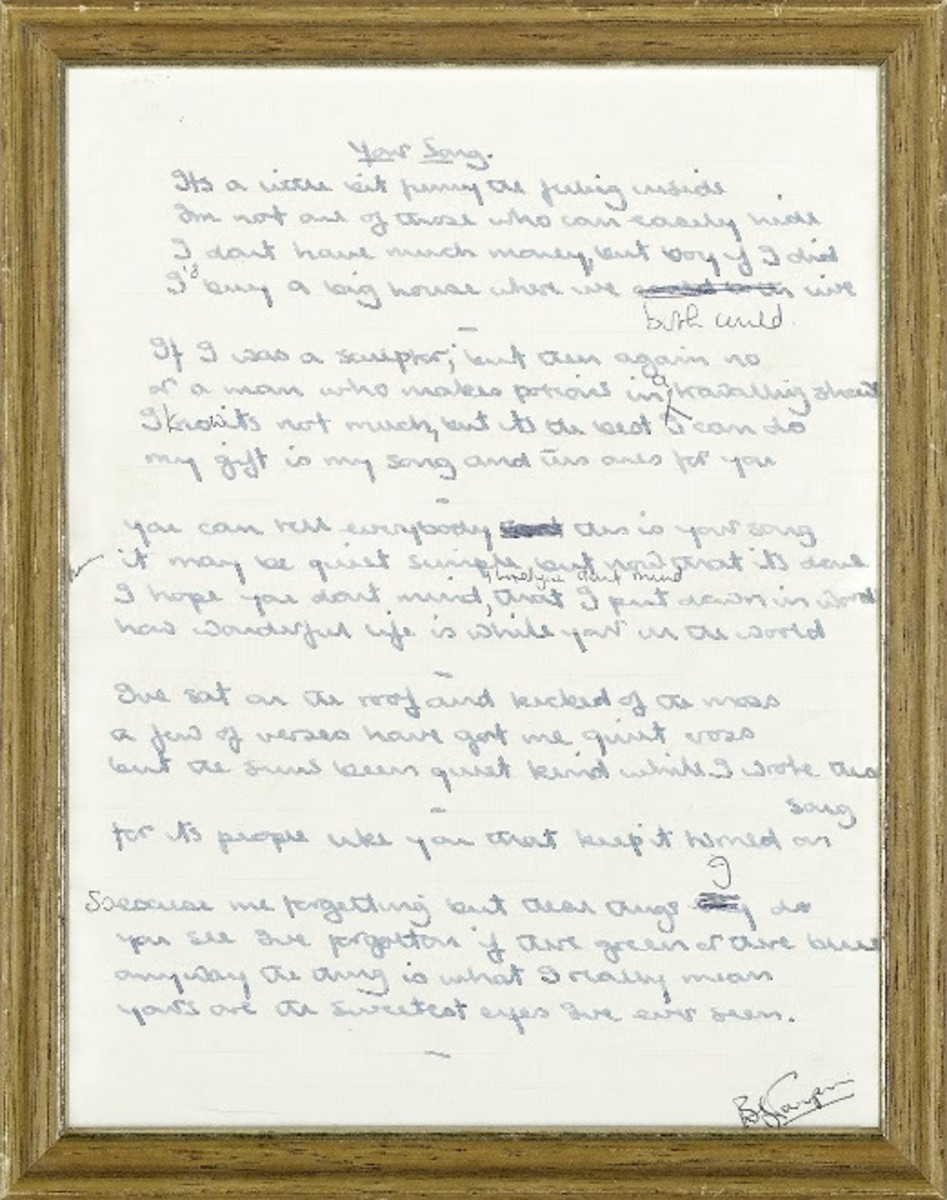In the image, there is a framed, handwritten page displayed prominently. The frame is a rectangular, brown wooden frame standing vertically. Inside, the paper appears aged and somewhat worn, giving it an antique feel. The top of the page is titled "Your Song," with both words underlined. The content underneath is difficult to decipher due to the faded and ornate cursive script. The text begins with the phrase "It's a little bit funny," which suggests that these are the original lyrics to the song "Your Song." Throughout the page, there are visible corrections—words scratched out and rewritten below them. At the bottom of the page, there is a cursive signature starting with the letter "B," though it remains mostly illegible because of the intricate script. Despite the challenge in reading the text, the neatness and care in the handwriting are evident, indicating the significance of preserving this piece in a frame.